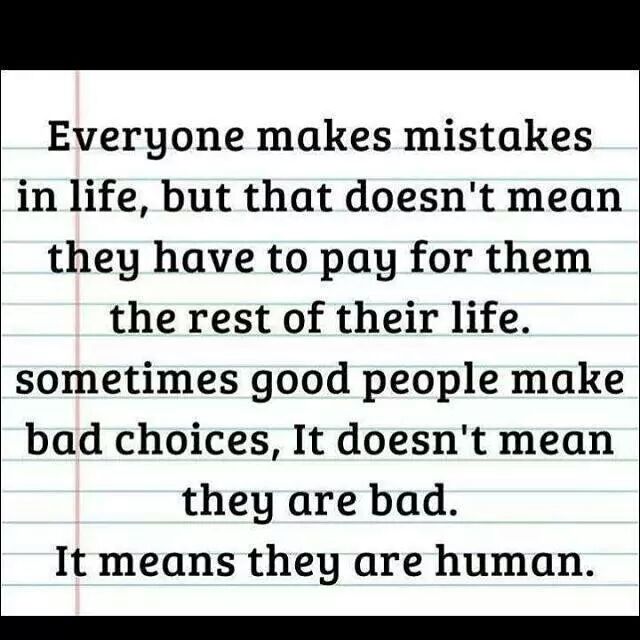The image depicts a printed note on a piece of notebook paper, bordered on the top and bottom by solid black bars. The notebook paper itself is classic white, lined with horizontal blue lines, and features a vertical red margin line on the left. The note spans eight lines of black text, each line of text corresponding to a blue line on the paper, with empty spaces between each. The text reads, "Everyone makes mistakes in life, but that doesn't mean they have to pay for them for the rest of their life. Sometimes good people make bad choices. It doesn't mean they are bad. It means they are human." However, this text contains several grammatical errors.